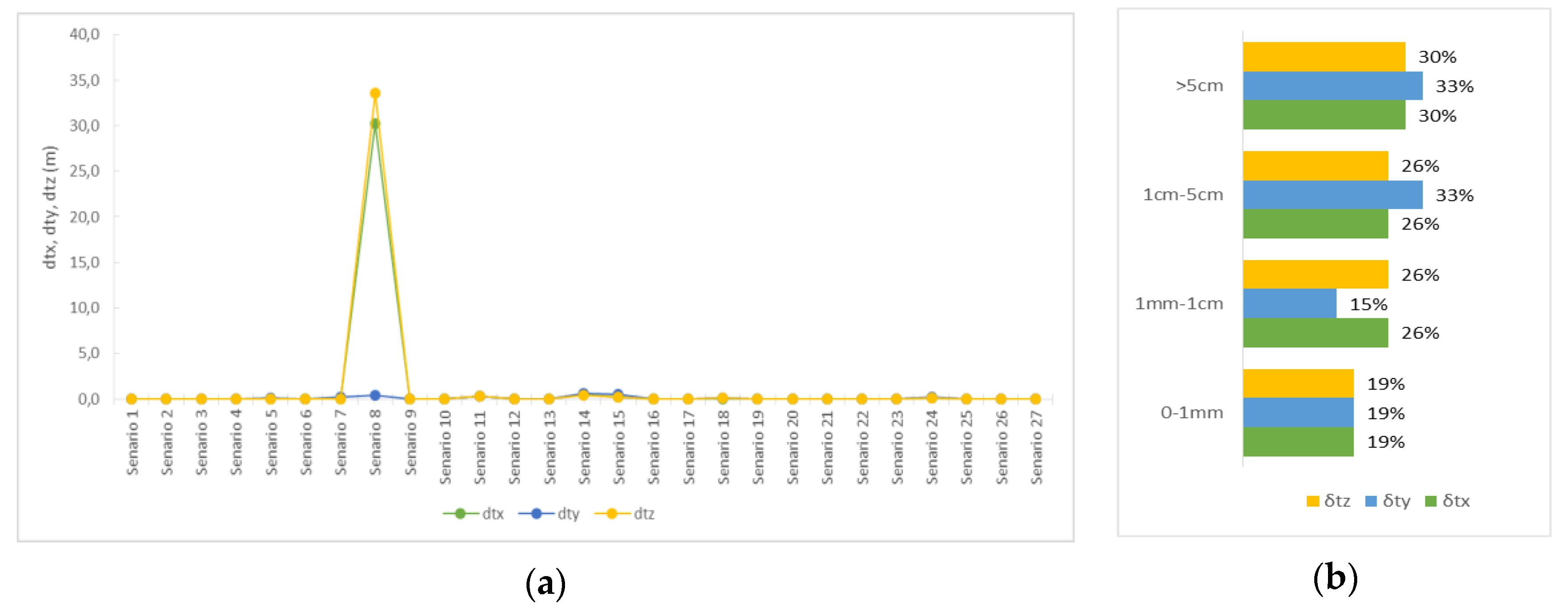The image consists of two distinct charts: Chart A on the left and Chart B on the right. Chart A is a line graph showing three distinct data lines: a yellow line (DTZ), a green line (DTX), and a blue line (DTY), plotted against two axes. The y-axis is labeled "DTX, DTY, DTZ (M)" and ranges from 0.0 to 40.0. The x-axis features scenarios numbered sequentially from 1 to 27. Notably, the DTY (blue line) exhibits significant peaks; at Scenario 8, it reaches approximately 30, and another substantial peak occurs up to 34. 

Chart B is a bar graph divided into four segments based on size categories: greater than 5 centimeters, 1 centimeter to 5 centimeters, 1 millimeter to 1 centimeter, and 0 to 1 millimeter. Each segment compares percentages for yellow (STX), blue (STY), and green (STX) bars. The distribution is as follows: for greater than 5 centimeters, yellow is 30%, blue is 33%, and green is 30%. For 1 centimeter to 5 centimeters, yellow and green are both 26%, while blue is 33%. For 1 millimeter to 1 centimeter, yellow and green are both 26%, and blue is 15%. Finally, for 0 to 1 millimeter, all colors are equally divided at 19%.

Overall, the graphs provide a detailed comparison of the distribution and variance of data across different scenarios and size categories, highlighting key peaks and proportional differences.